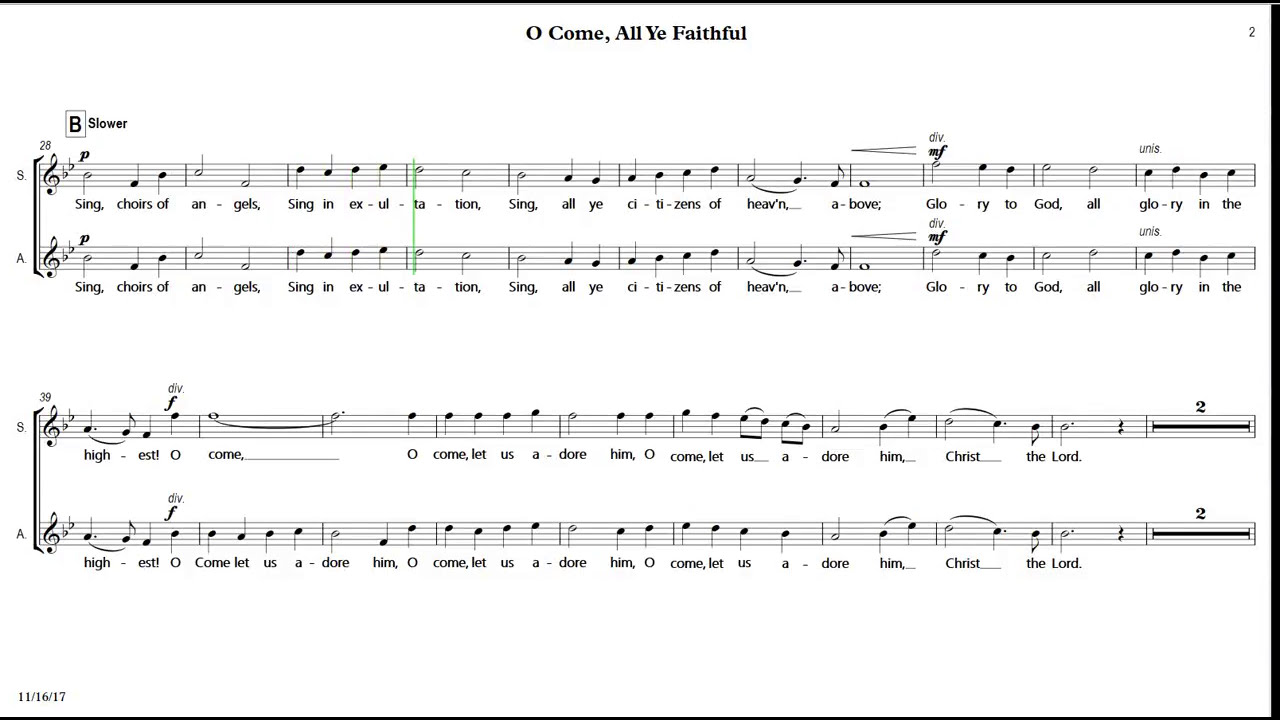This image features a sheet of music on a white background with a black edge border in the upper right corner. At the top center, in black text, it reads "O Come, All Ye Faithful." Positioned in the upper left corner, bold lettering indicates the key of B and the tempo "slower." The sheet contains six bars of music, with a treble clef on the left side. The musical notation includes both soprano and alto lines, allowing for both vocal and instrumental rendition. The lyrics are interspersed within the musical notes and read: "Sing, choirs of angels, sing in exultation, sing all ye citizens of heaven above, glory to God, all glory in the highest. O come, O come, let us adore Him, Christ the Lord."